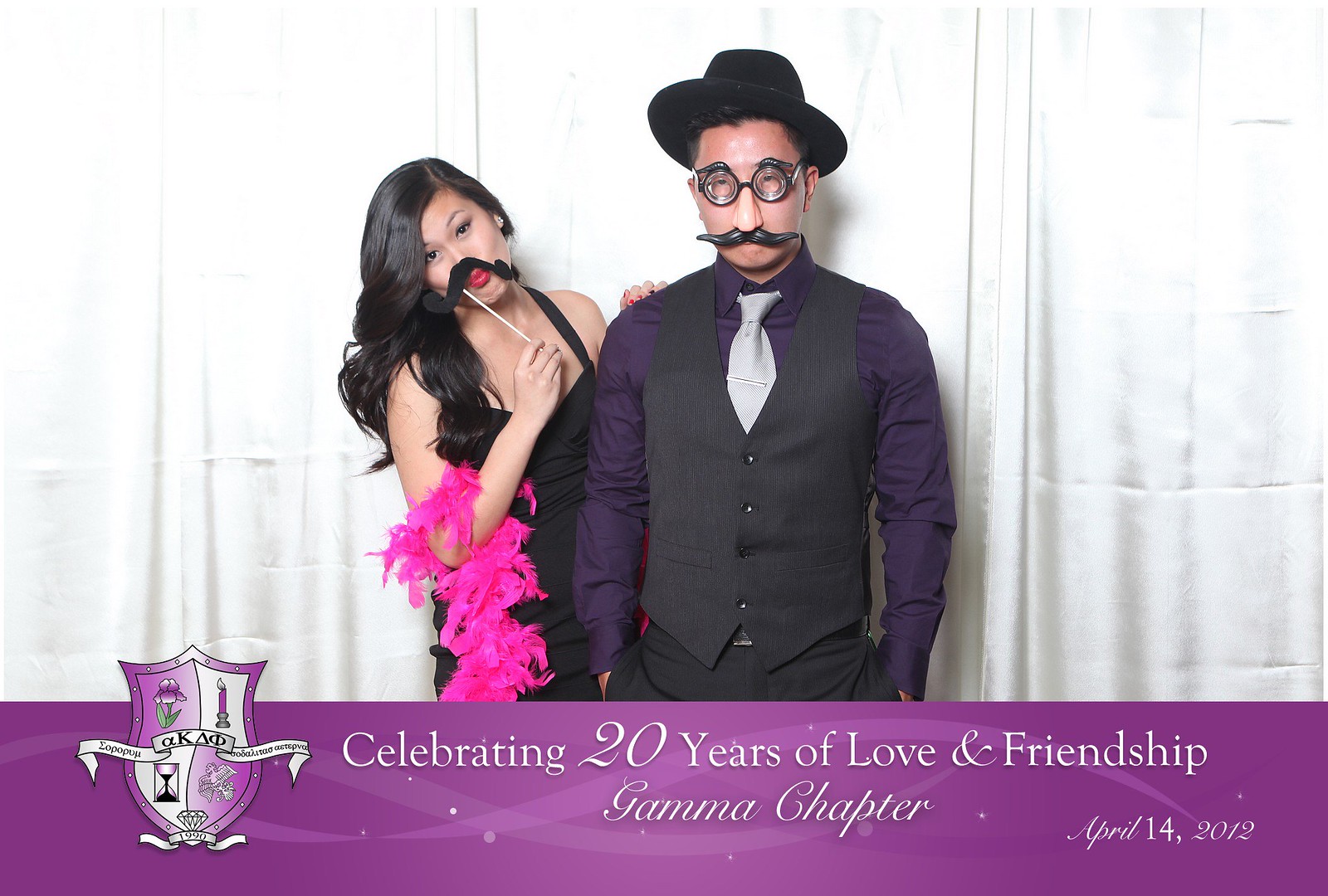In front of a white curtain, a couple strikes a playful pose for a photo booth picture, commemorating a special event. On the right, the man sports a quirky ensemble with a black vest and pants, a silver tie over a purple dress shirt, and a black bowler-like hat. His comical accessories include oversized plastic glasses with a fake nose, large fake mustache, and additional fake eyebrows. To his left stands a woman in a sleek black dress, her dark black hair cascading over her shoulders. She accessorizes with a bright purplish-pink feather boa draped over her elbow and holds up a fake mustache on a stick to her red lips. Both are engaged in the playful spirit of the moment. At the bottom of the image, white lettering against a purple background reads, "Celebrating 20 Years of Love and Friendship, Gamma Chapter, April 14, 2012". To the left of the text, there is a symbol or seal, presumably representing the Gamma Chapter.